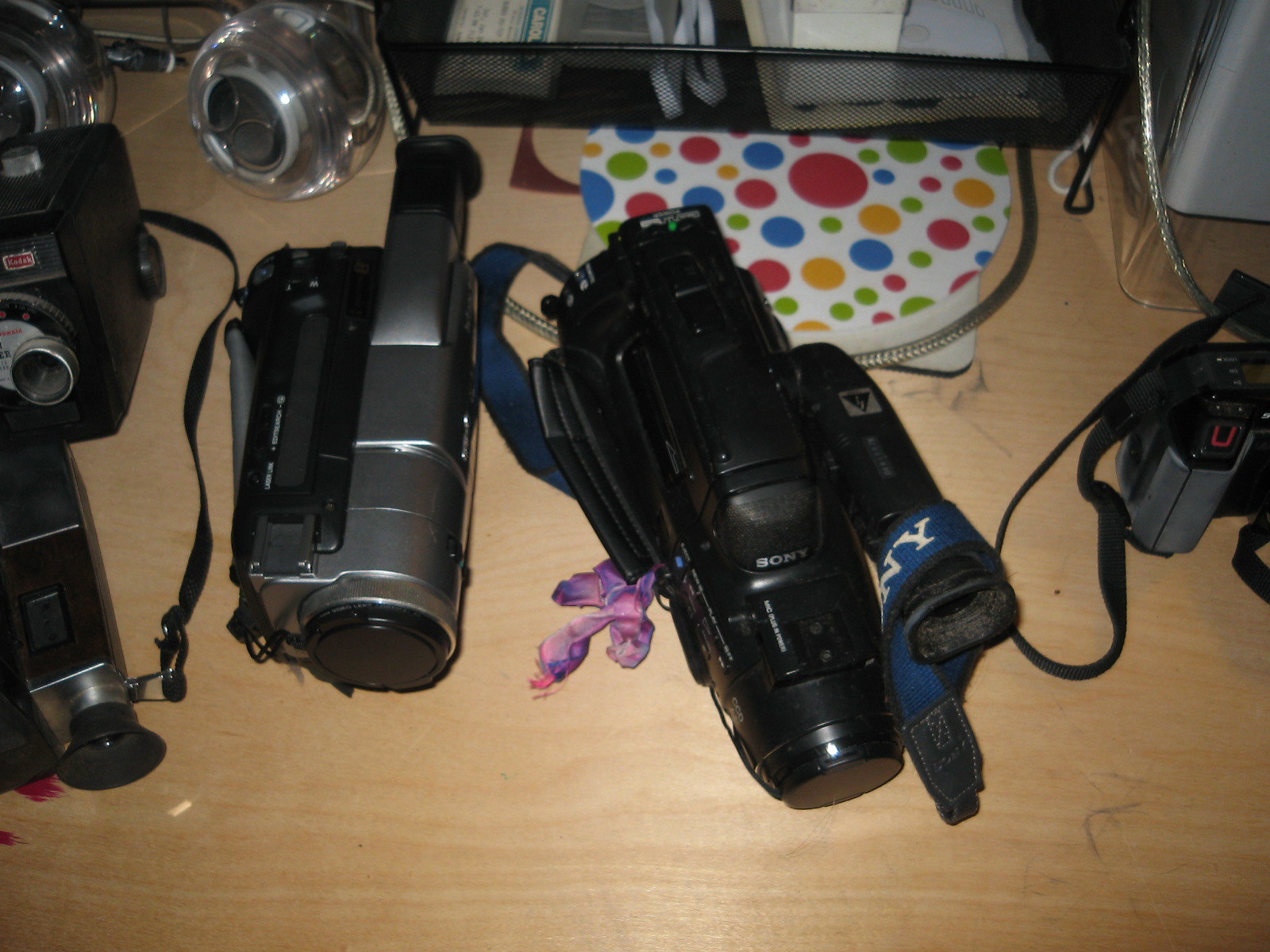This image captures a collection of camera equipment arranged on a light brown wooden desk. At the center sits a black, long-shaped Sony camcorder, distinguishable by its purple ribbon tied to the side. To the right of the Sony camcorder, there's a gray, black, and red camera featuring a thin black strap and a visible black screen and handle. On the left, a large silver camera with a prominent lens is positioned next to another partially visible camera at the far left. In the background, a circular white mat adorned with colorful polka dots in green, orange, blue, and red adds a vibrant touch. Additionally, a black basket holding various items and a couple of gray circular objects are situated above the mat.